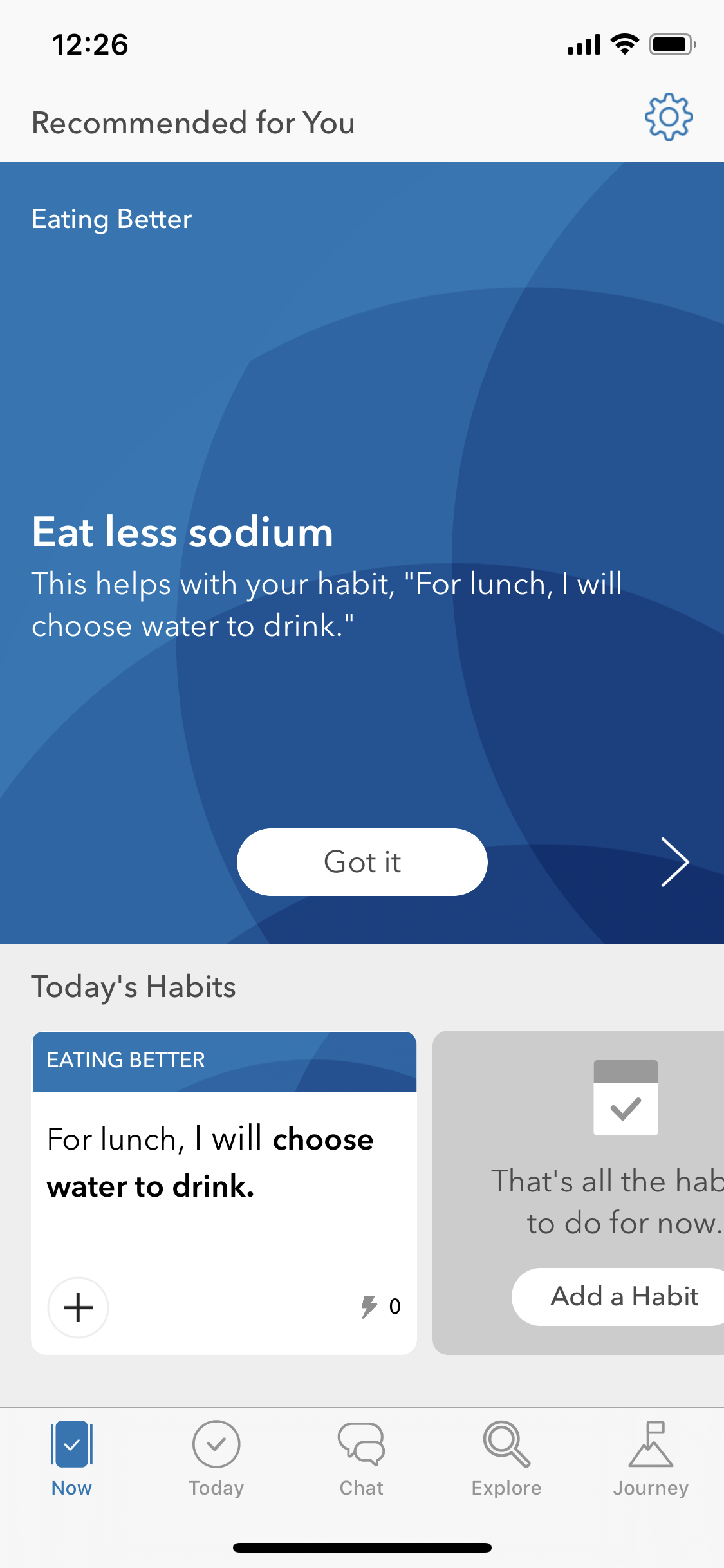This image is a screenshot from a mobile app designed for meal planning, dieting, or tracking healthy eating habits. At the top of the screen, there is a "Recommended for You" section, accompanied by a blue gear icon on the right, which likely represents the settings button. Below this section, a blue box labeled "Eating Better" occupies the top left, containing a central message: "Eat less sodium. This helps with your habit. For lunch, I will choose to drink water." A white bubble button labeled "Got it" is positioned underneath this text.

Further down, another section titled "Today's Habits" appears, featuring a blue and white box with the repeated message: "For lunch, I will choose water to drink." To the right of this box, there is a statement indicating, "That's all the habits to do for now." Additionally, a button to "Add a habit" is available for users to customize their tracking.

At the bottom of the screen, navigation buttons for "Now," "Today," "Chat," "Explore," and "Journey" are visible, offering various functionalities within the app. The layout and options within the app emphasize organization and ease of use, targeted at promoting healthier eating habits and lifestyle changes.